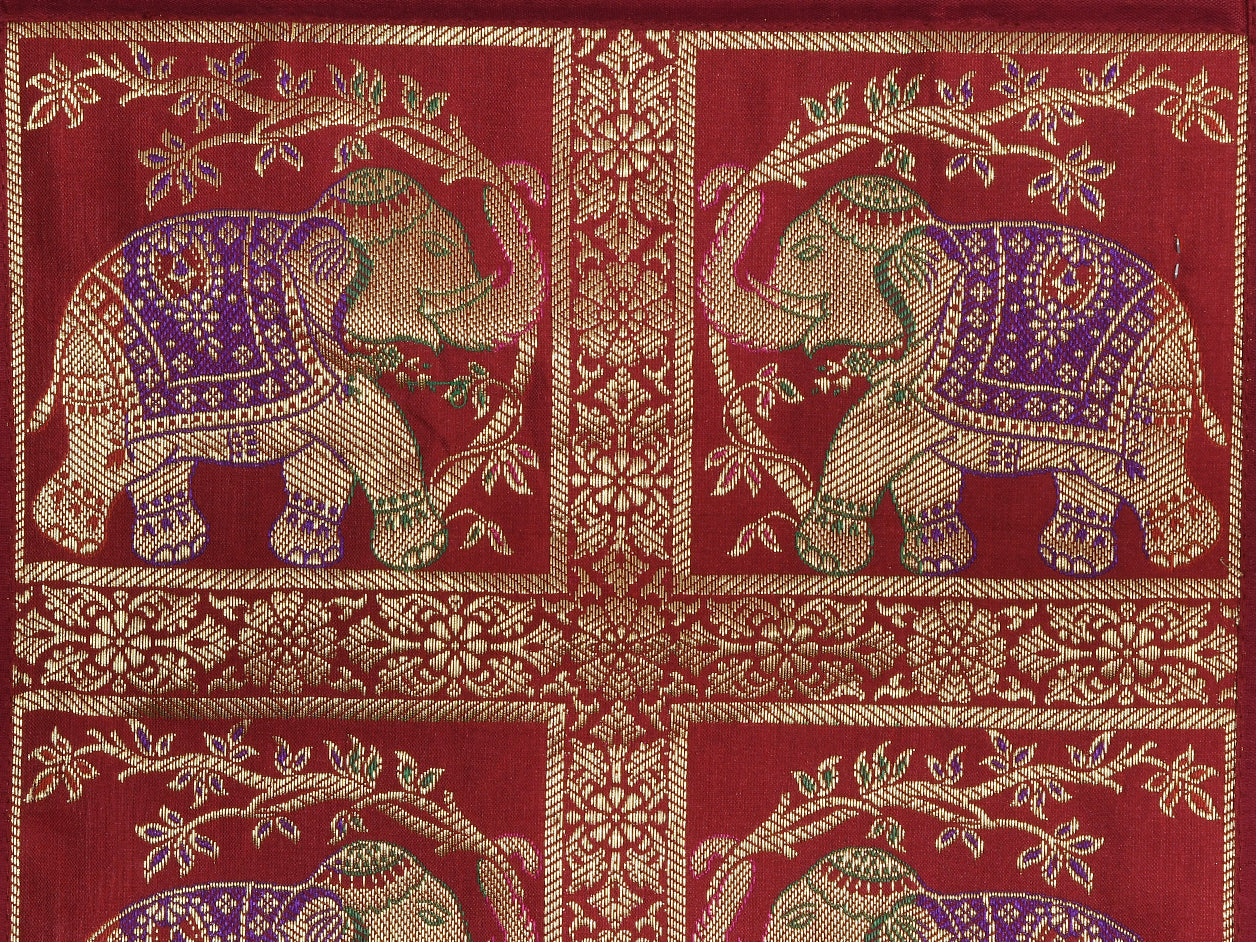This image depicts a detailed Indian tapestry that features a rich maroon background adorned with intricate gold embroidery. The tapestry is divided into four sections by an ornate gold brocade, each section showcasing pairs of elephants facing each other. The elephants, rendered in a base gold color, carry substantial branches with green leaves in their trunks. Each elephant is adorned with a vibrant ensemble, including purple and gold draped cloths with a central red symbol encasing a gold diamond. They wear ornate headgear accented with red, green, and maroon hues, and each elephant has prominent tusks, suggesting an ancient and traditional aesthetic. The tapestry's border is embellished with delicate gold motifs against the maroon backdrop, enhancing its vintage and ornate appearance. This celebrated artwork portrays a harmonious repetition of design and color, seamlessly blending the elements of Indian culture and textile craft.